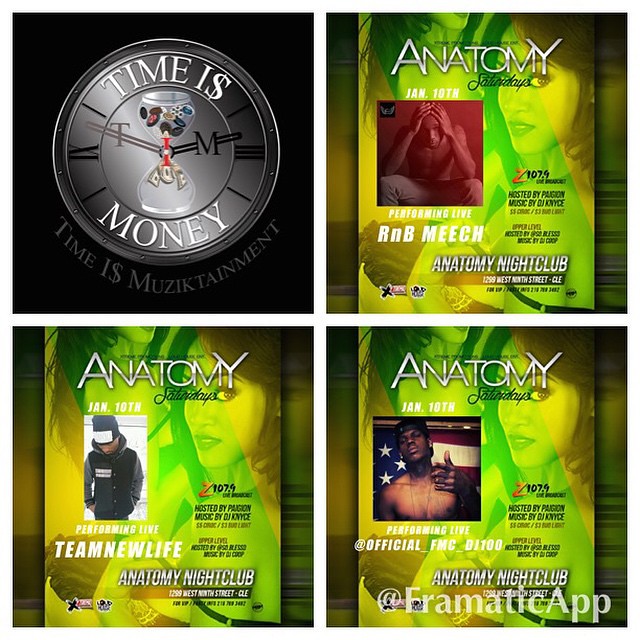The image is a promotional flyer divided into four equal quadrants by white lines, each spotlighting a different aspect of an event at the Anatomy Nightclub. The top left quadrant features an illustration of an hourglass with money flowing through it, alongside a clock, both accompanied by the text "Time is Money" and "Time is Musictainment." The top right and the lower two quadrants showcase images related to the nightclub performances. Each of these three sections has a background image of a woman, with the top right quadrant including a man with his hands on his head, the bottom left displaying a performer named "Team New Life" in a hoodie, and the bottom right featuring a topless man with an American flag behind him. Prominent text highlights event details such as "Anatomy Saturdays," "Jan 10th," and the performers "R&B niche," "Team New Life," and "Official_FMC_ D/100." The color palette includes red, white, blue from the flag, as well as splashes of black, gray, green, and yellow, underscoring the vibrant yet structured promotional style of the nightclub event.